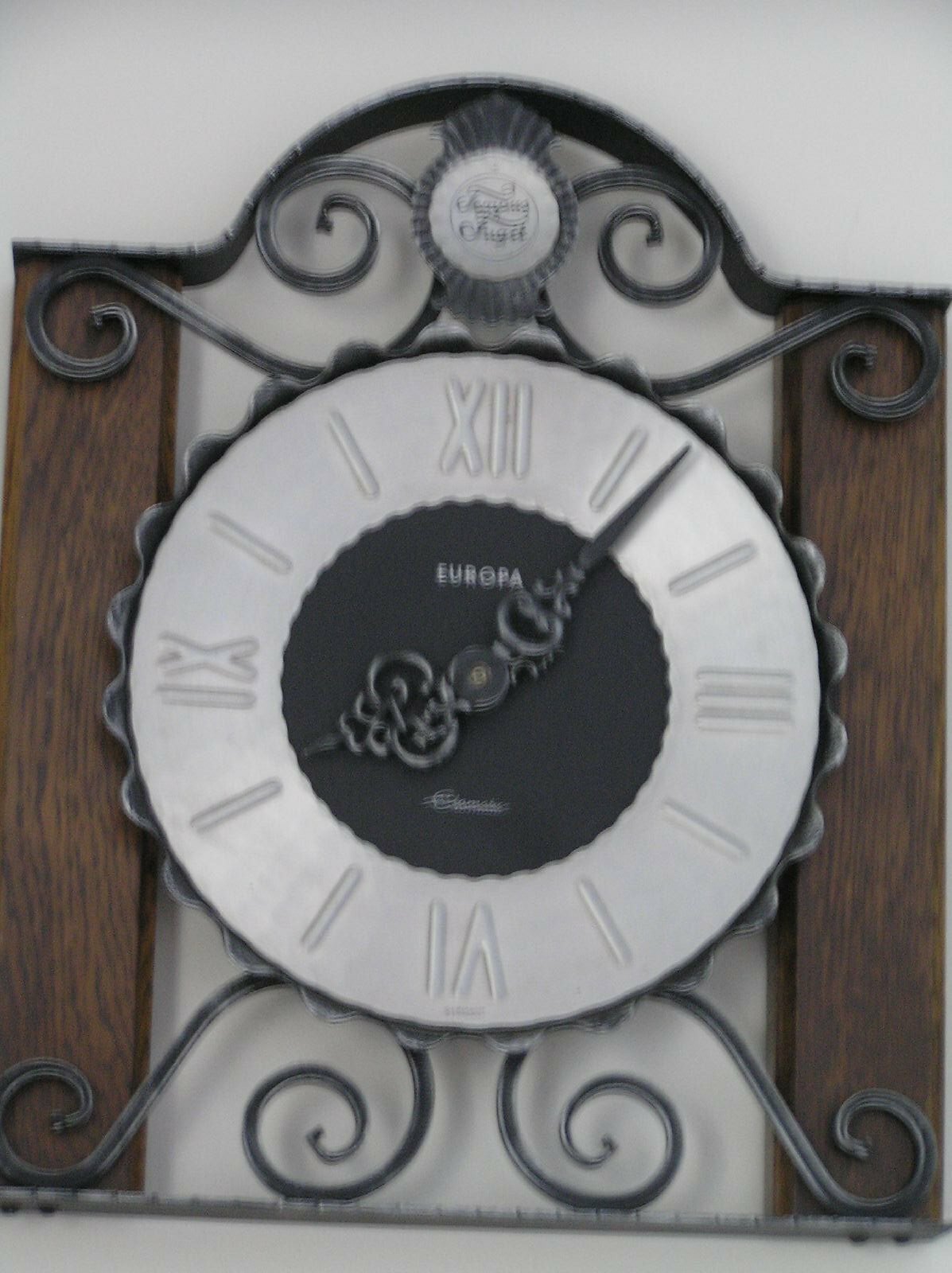The image features a prominent, gigantic clock face branded with the word "Europa" in white letters at its center. The clock is circular with an aesthetically pleasing set of hands and Roman numerals marking the hours. The face of the clock is encased in a metallic, silverish frame, complemented by several ornate, wavy metal motifs. A distinct black circular border outlines the clock. The background wall is flat and white, adding to the clock's prominence, with attached dark brown wood panels vertically flanking the left and right sides. Above the clock, a ribbon-like structure in black and silver stretches across, though the text on it is not legible. This elaborate design provides a striking and detailed focal point in the image.